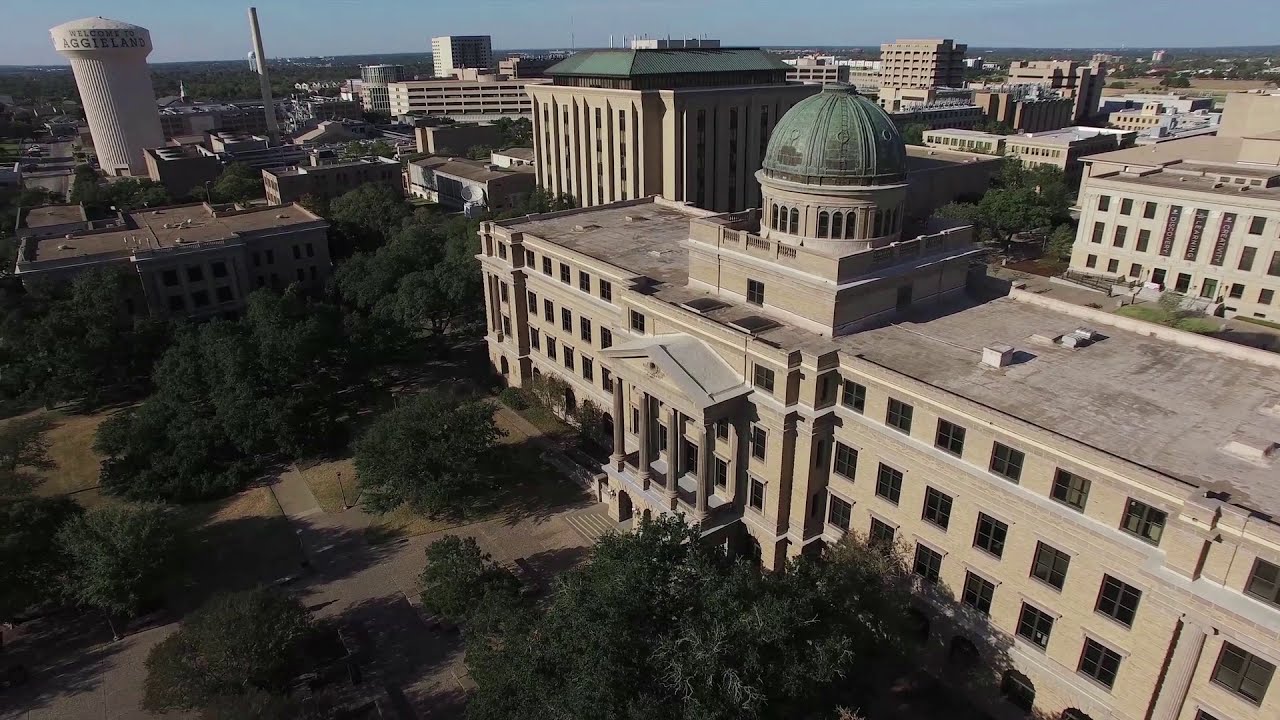The image captures an aerial panoramic view of a city, centered on a large, prominent building that appears to be City Hall or a state capital. This focal building features a distinctive green copper domed rotunda atop a tan, likely concrete structure with four floors and possibly a fifth including the ground floor. The entryway is characterized by four substantial columns supporting an A-frame roof, which is equipped with solar panels and vents. Surrounding the entry are laid pavers or bricks and various large, green bushy trees. To the left, a secondary building with a slightly higher flat copper roof is visible, presumably containing classrooms. A water tower stands prominently to the left. In the background, there’s a dense arrangement of buildings in off-brown and grayish tones, with a patch of blue sky stretching across the horizontal axis, adding a serene backdrop to the bustling cityscape below.